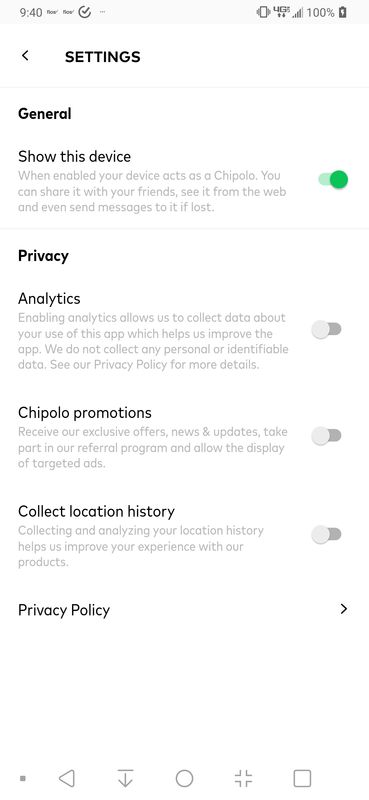The image captures a smartphone screen displaying its settings menu. The time shown is 9:40 AM, and several status icons, including a fully charged 100% battery and three additional indicators, are visible at the top of the screen. As we look further down, the settings are organized under the "General" category.

A notable section titled "Show This Device" features a slider that is toggled on, enabling the function that turns the device into a Chipolo. This feature allows the device to be shared with friends, located via the web, and receive messages if lost. The subsequent settings include "Analytics" and "Chipolo Promotions," both of which have their sliders turned off. The "Collect Location History" option is also disabled. At the bottom, there is a "Privacy Policy" entry with a right-facing arrow indicating further information.